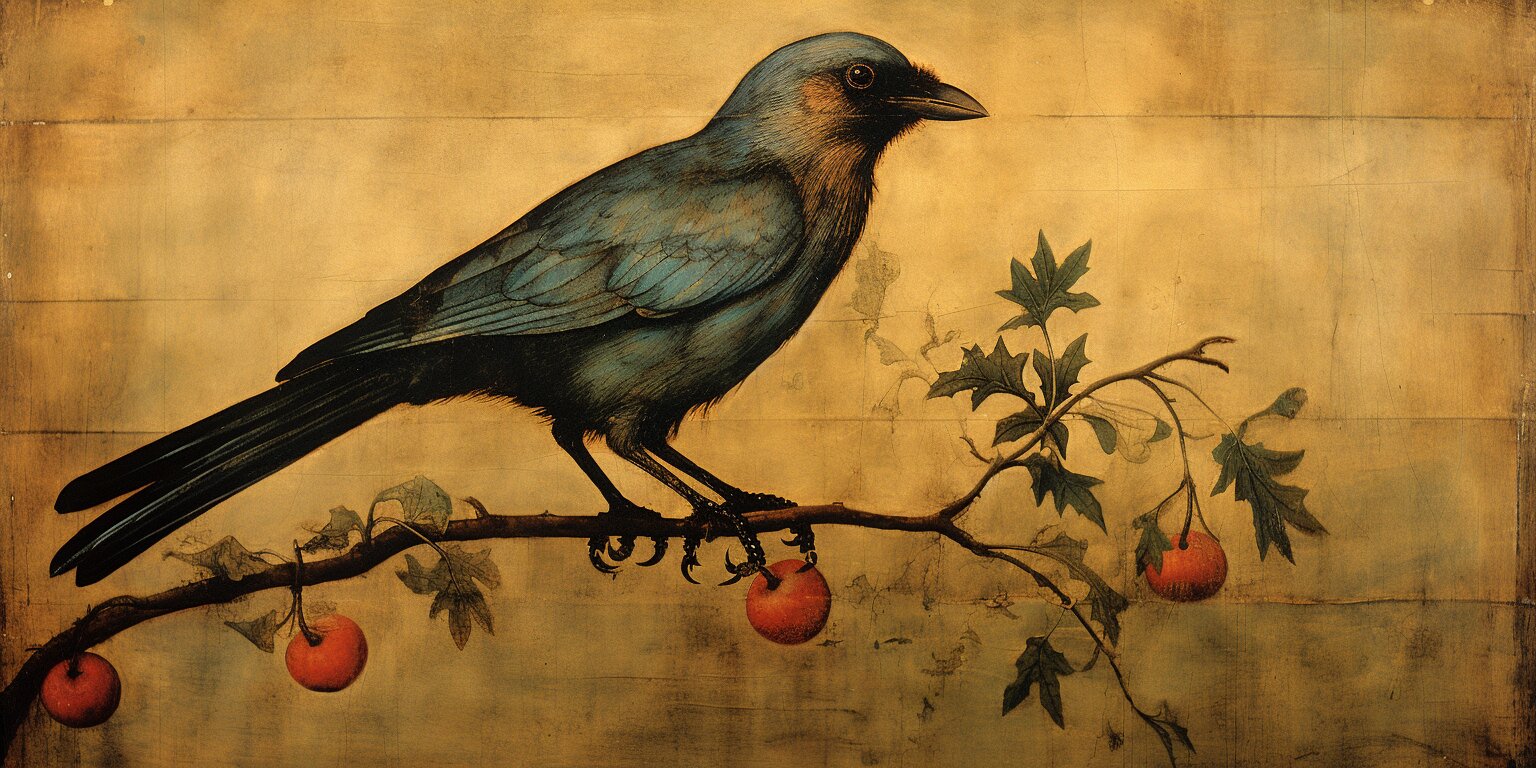This is a detailed painting of a blue bird perched on a thin branch of a tree. The bird, shown in a side profile, showcases a blend of blue tones with some orange and yellow hues near its face, and darker tail feathers. Its intricate details include beady black eyes and talons grasping the branch. The branch, adorned with green leaves, also has four colorful apples—orangey-red in hue—dangling from it. The background features a weathered, old appearance with brownish-yellow and beigey brown hues, adding texture and depth to the scene, reminiscent of a worn wall. The painting is on paper that looks yellowed, almost like it's coffee-stained, enhancing the vintage feel of the artwork.